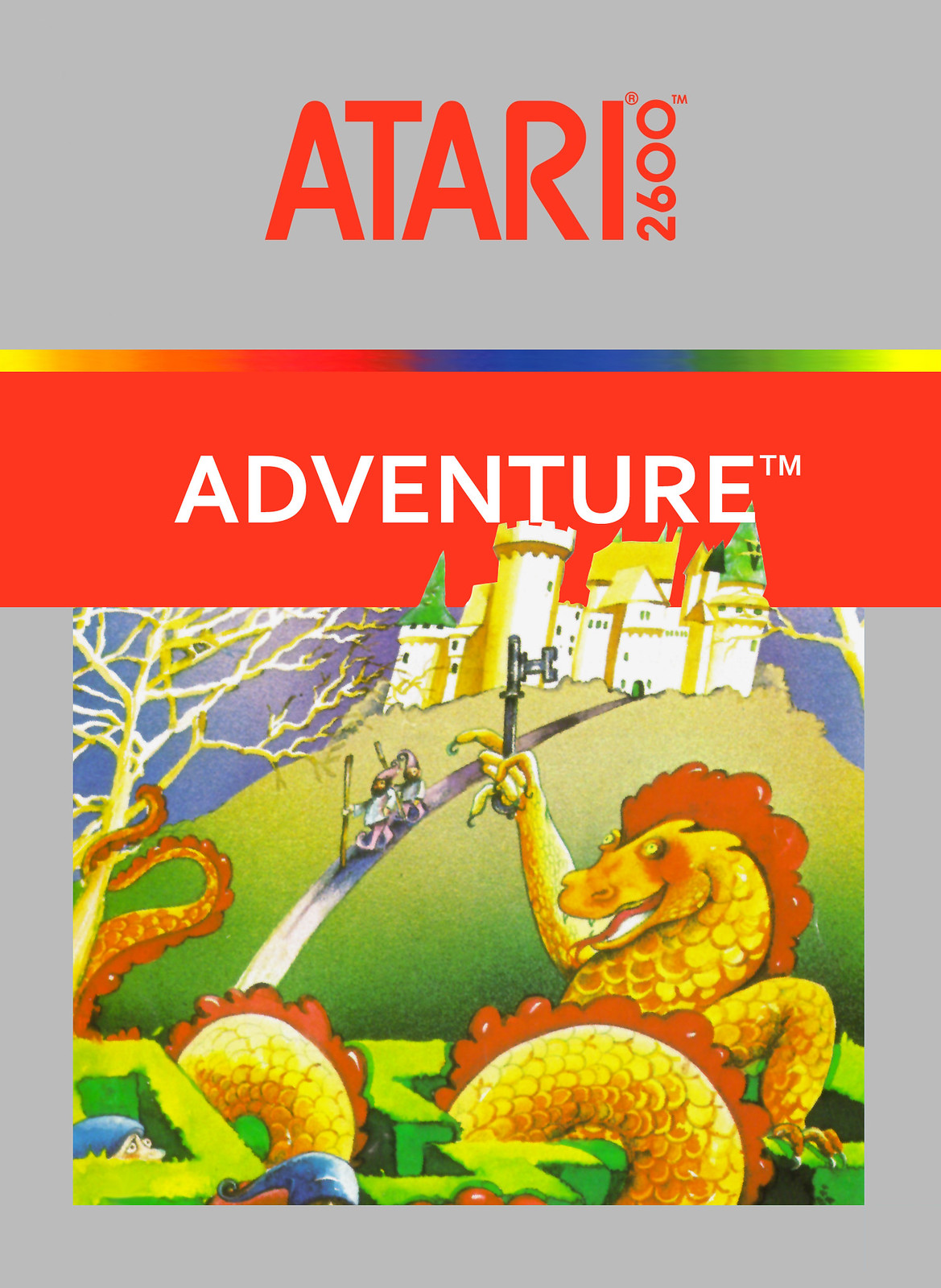This image appears to be the cover of an old game for the Atari 2600 system titled "Adventure™". The dominant color of the cover is grey, with the "Atari 2600" label prominently displayed. In a vivid, cartoonish art style, the scene features a castle with multiple turrets standing majestically in the background. A vibrant red and yellow dragon is depicted holding a vintage key, symbolizing access to a mysterious door. In the foreground, two men are seen walking away from the castle along a distinct pathway. Adding to the scene, a tree stands prominently, enhancing the medieval and adventurous atmosphere of the game cover.